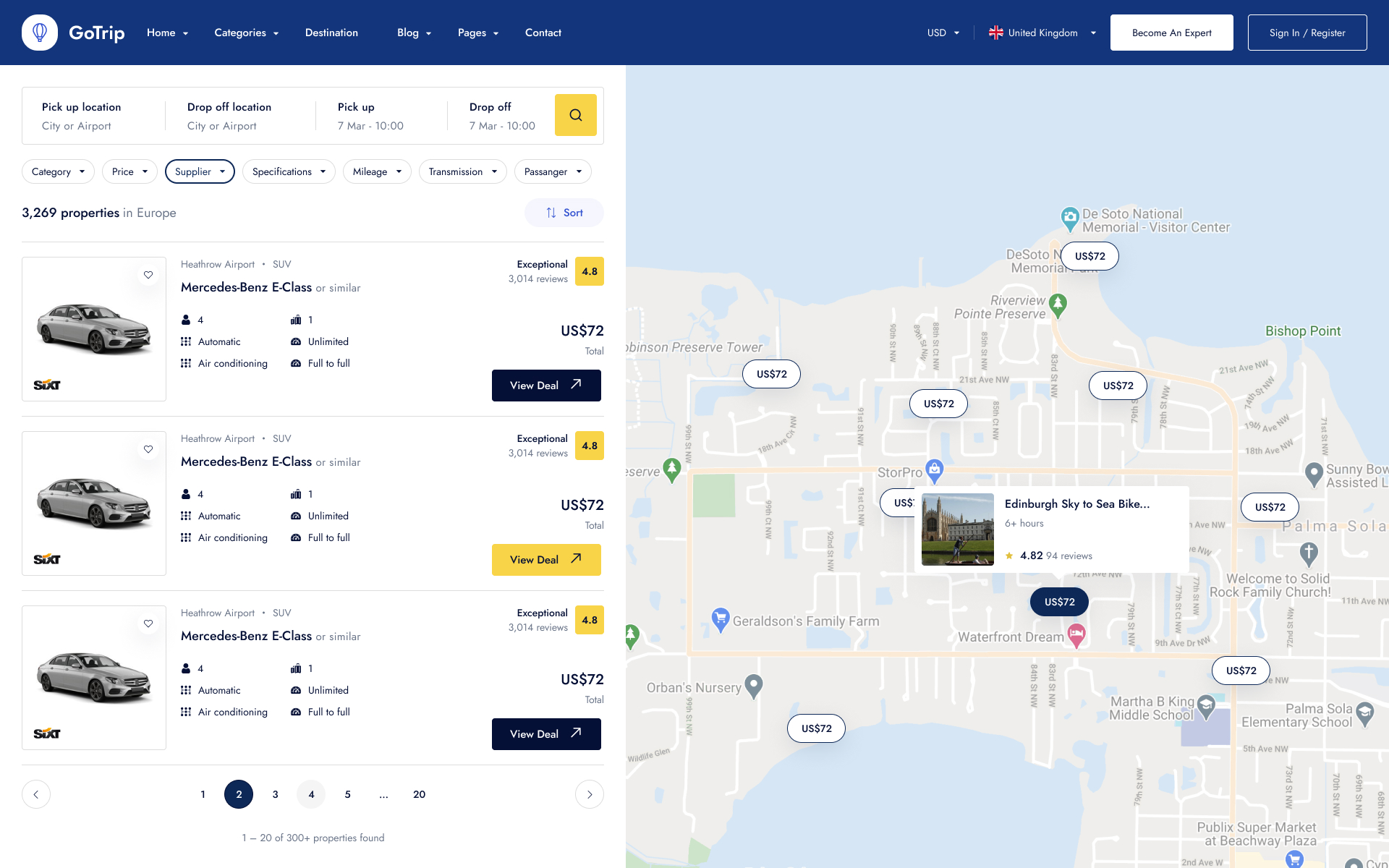Here is a detailed caption for the image of the GoTrip website:

---

A screenshot of the GoTrip website, showcasing its user-friendly layout and design. The top of the webpage is dominated by a sleek navy blue navigation bar with white lettering. For users in the United Kingdom, a red, white, and blue-themed display, complete with the United Kingdom flag preceding the word "United," indicates the selection for the region.

On the left side of the screen, there's a comprehensive selection of rental cars available, each detailed with price and pickup location information. On the right, an interactive map outlines the area of interest, highlighting the exact locations where rentals can be picked up. 

A prominent feature on the page is a detailed view of an Edinburgh Sky to Seabike location, designed to provide users with a closer look at specific rental options. Additionally, three available cars are prominently displayed - all Mercedes-Benz E-Class or similar models, ready for pickup from Heathrow Airport, each priced at $72. These vehicles appear in shades of white or light grey, emphasizing their luxurious and pristine condition.

---

This caption captures the essential elements of the website, providing a clear and detailed description of its features and layout.